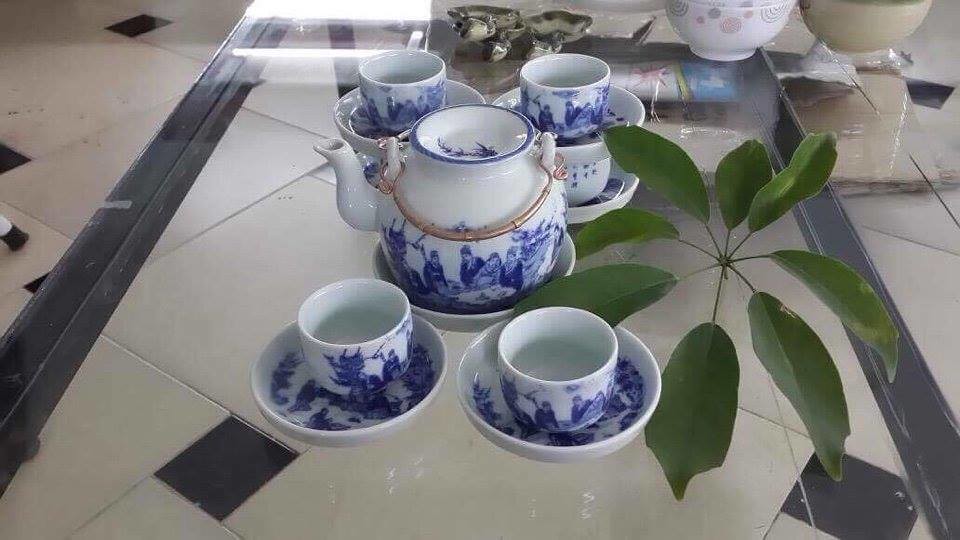This photograph showcases an elegant Asian-inspired tea set arranged on a table with a surface of white tiles featuring blue insets and a blue border. The tea set includes five cups and saucers, all without handles, and a central teapot equipped with a bamboo-style handle. Each teacup, saucer, and the teapot showcases intricate blue illustrations of Asian figures on a pristine white background. Adding to the scene, a green house plant with lush leaves sits to the right, casting a natural element against the reflective, tiled tabletop. The setting suggests a serene ambiance possibly intended for showcasing or selling this ornate tea set. Additionally, in the background, a few more bowls bearing similar blue and white designs are visible, some with gold accents and others featuring red and green patterns.